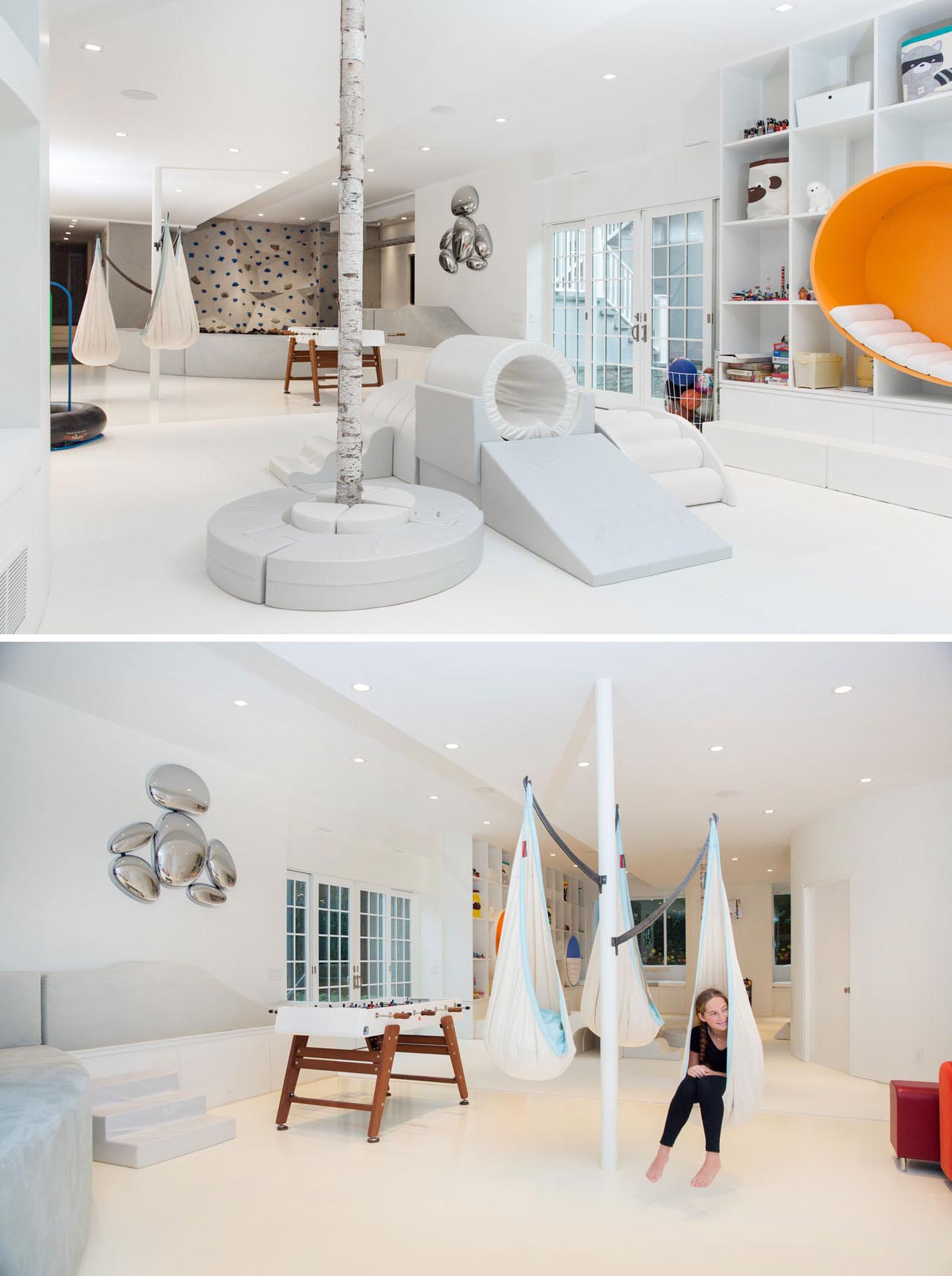The image consists of two separate photographs showcasing the modern interior of a home, with both pictures capturing different angles of the same white-themed room. In the top photograph, the room features sleek, all-white floors and walls adorned with polka dot patterns. Central to this space is an intriguing white structure that resembles a play area, complete with a white tree trunk or pole and a series of gymnastic cushions forming a tunnel and steps, possibly designed for children or pets. To the right, the room boasts large white cabinets filled with boxes and toys, with cubbies hosting cozy orange pillows. A door with a window leads to another area, and the backdrop features a metallic statue design made up of oval shapes reminiscent of a human figure.

The bottom photograph provides a view of the same room from a different perspective. Here, there are multiple white hammock chairs attached to a pole running from the floor to the ceiling. A foosball table is also present, contributing to the playful atmosphere. On one of the hammock chairs, a young girl dressed in black, with light brown hair braided to the side, is seated, adding a touch of life to the pristine setting. The room is marked by its continuity in design elements, including the striking metallic artwork on the walls and recurring gymnastic cushions, further emphasizing its modern and minimalist aesthetic.